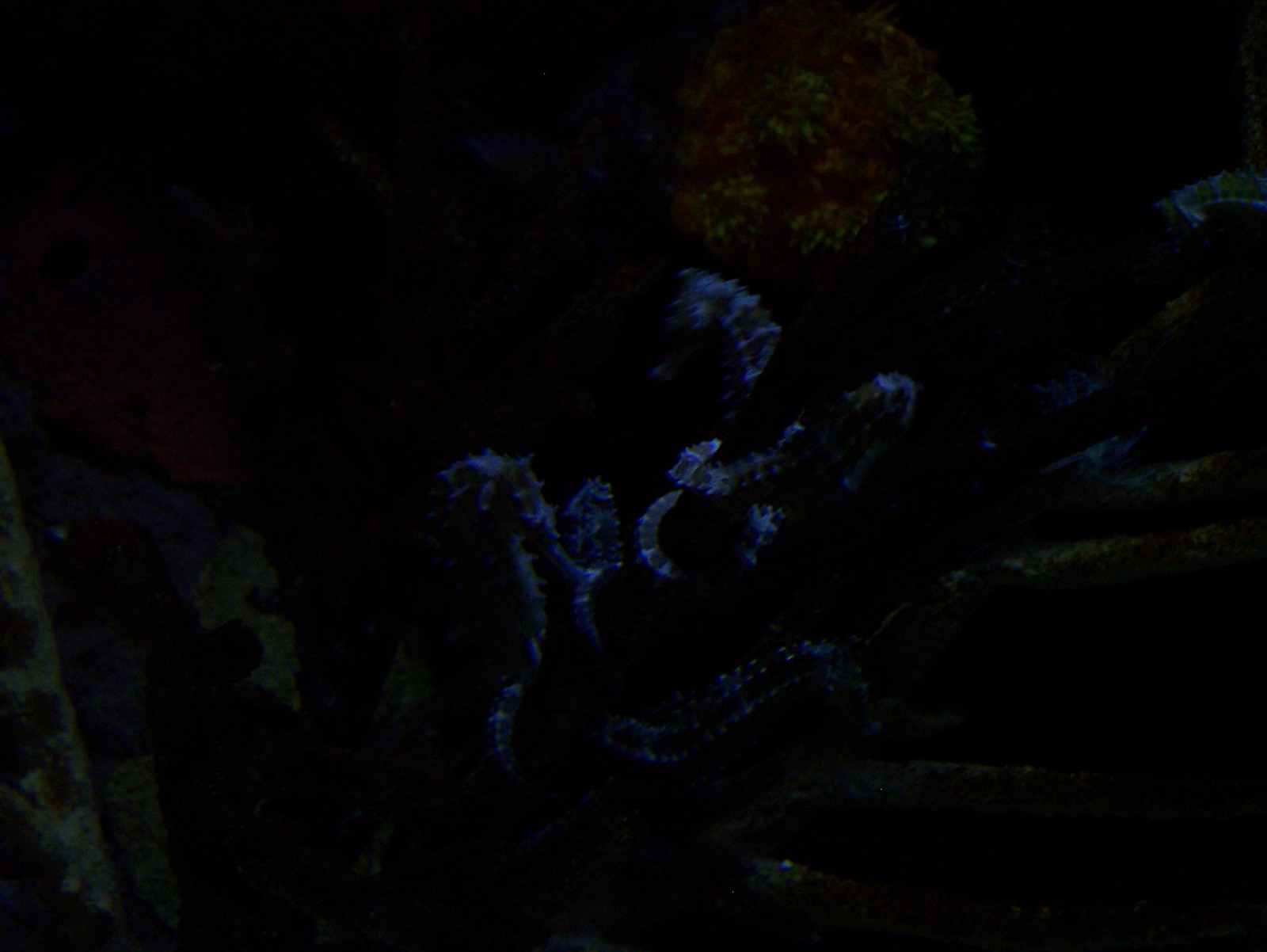This image is primarily enveloped in darkness, making detailed observation challenging. At the center, faint light reveals rocks or coral with a bluish tint, suggesting an underwater scene. Outlines of two seahorses become discernible, characterized by their distinctive horse-shaped heads and slightly armored bodies, glowing faintly amidst the darkness. Some sparse vegetation can be seen in the background, adding a touch of brown and green hues to the predominantly black canvas. The scene also features spiky, pointy structures resembling corals, but their exact forms are hard to distinguish due to the low lighting. Overall, while the image's specific details are elusive, the interplay of dim light and shadow suggests an underwater cavern or reef shrouded in darkness.